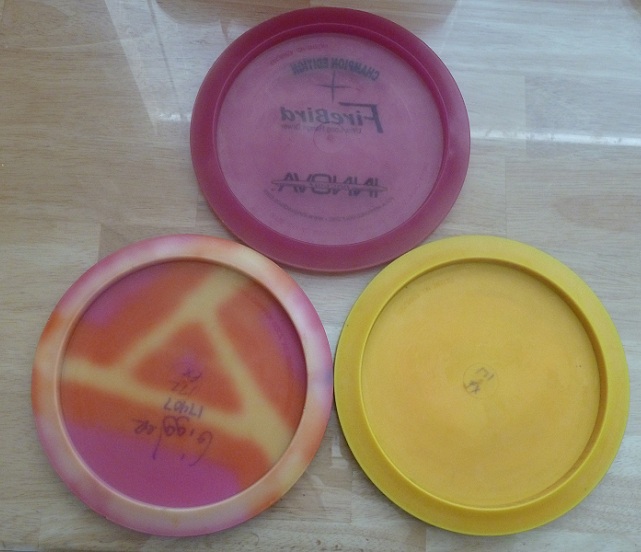The image features a close-up of three frisbees arranged in a triangular formation on a glossy light brown hardwood floor. The frisbee at the top, which has a vibrant red color and bears the logo "Frisbee" and a partially legible company name that appears to be Avon or Avonnie, is upside down. On the right is a plain yellow frisbee, also flipped upside down. The bottom left frisbee displays a vivid mix of yellow, orange, and pink colors, reminiscent of a tie-dye pattern, and features an upside-down logo. All three frisbees are positioned such that their interiors, resembling small plates, are visible. The aerial perspective of the shot highlights the reflective nature of the floor and the distinct color variations of the frisbees.